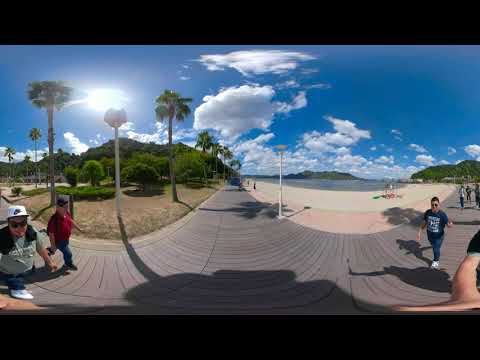The image depicts a sunny, tropical scene captured with a wide-angle or 360-degree lens, creating a slightly distorted, rounded view. The sky is a clear blue with scattered puffy white clouds, and the sun shines brightly from the upper left quadrant, casting a warm glow over the scene.

In the center of the image, a grayish cement boardwalk stretches across a vibrant landscape, appearing slightly curved due to the lens distortion. The foreground of the boardwalk features several individuals walking, clad in casual attire. One person is notable for wearing jeans, a dark t-shirt with white handwriting, and sunglasses. Another person is dressed in jeans, a t-shirt, sunglasses, and a baseball cap. Additionally, there is a person in jeans and a red polo shirt with a baseball cap. Most of the visible people on the boardwalk are donning jeans, short-sleeved shirts in various colors (green, red, blue), and sunglasses. 

To the left of the boardwalk, there are three tall palm trees and a variety of smaller shrubs, with a patch of dry brown grass leading to a lush green grove of trees in the background. To the right, the landscape transitions into a beachy area with sandy shores and sparkling water, extending to distant green hills. In the background to the right, several small groups of people can be seen strolling along the boardwalk and by the water, enjoying the picturesque and serene environment.